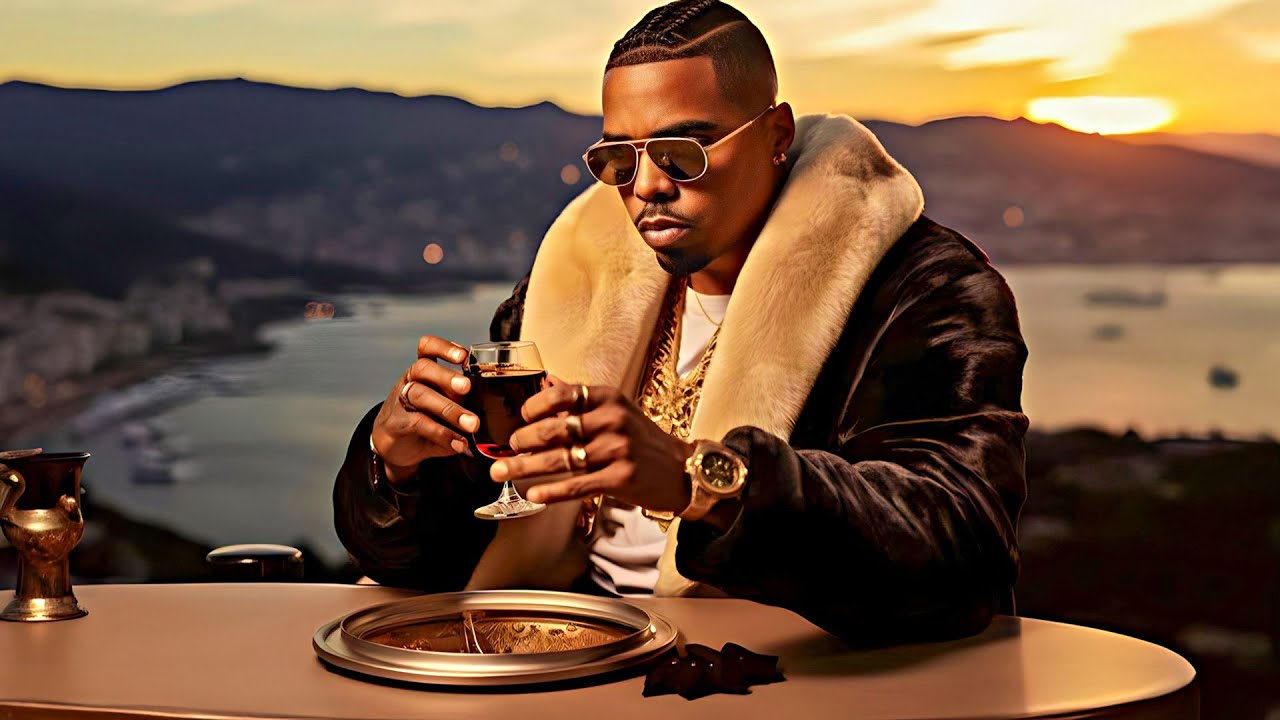A striking image captures a young Black man, likely in his twenties, exuding an air of opulence and sophistication. He stands adorned in a luxurious fur coat, its plush collar framing his face with an elegance that matches the gold chains draped around his neck. His right wrist is decorated with a gleaming gold watch and three ornate rings, while his left hand sports an additional ring. He holds a glass of wine with both hands, adding a touch of refinement to his ensemble. His eyes are hidden behind stylish sunglasses, and his meticulously groomed hair complements his overall polished appearance. In the background, a serene beach scene at sunset unfolds, casting a sublime glow over the entire composition. The photo, marked with the label "FIVO" in the bottom left corner, evokes a sense of grandeur, blurring the lines between reality and digital artistry, leaving one to ponder if it’s an authentic capture or a masterful piece of AI-generated art.